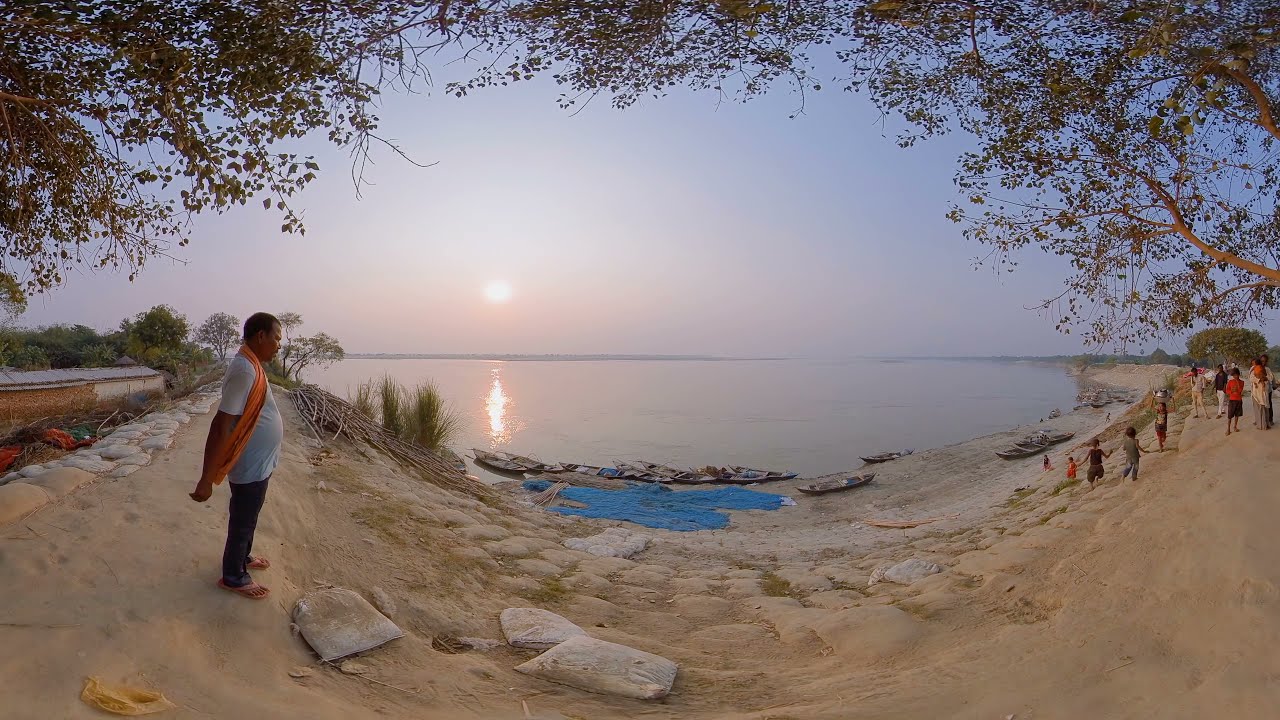The photograph captures a serene riverside scene during sunset. The foreground features a stretch of rippled sand curving gracefully from the left to the right of the image, possibly due to natural formation or a photographic distortion. A man stands to the left, slightly elevated on the sand, dressed in a white t-shirt, black pants, with an orange sash or scarf draped over his shoulder, and wearing orange sandals. He gazes towards the water with his hands behind his back.

Below, scattered around a small beach area are white rocks and several boats and canoes, some resting on the sand and others near the water’s edge. Blue plastic sheeting and sandbags, possibly part of a seawall or water defense, can be seen trailing down some steps leading to the riverbank.

To the right, a group of children and adults occupies the steps and sandy slope, with the children playing and holding hands as they move uphill. The background reveals sparse, green-leaved trees arching over the scene and framing the sky, which showcases the setting sun descending towards the horizon. The sky is a mix of soft blues and vibrant oranges, casting a golden reflection across the silvery water. The tranquil river, which is silverish and reflective, stretches towards faint land in the distance, completing this picturesque and peaceful setting.